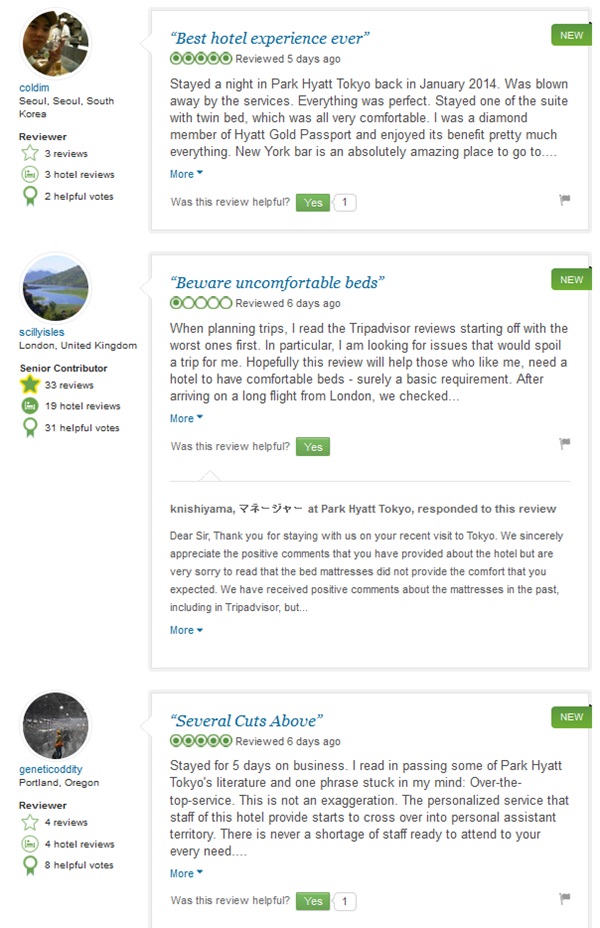This image depicts a review site showing three user profiles with detailed feedback about their hotel experiences. Each profile is represented by a circle with the user's information and review.

1. **User: Coldim (COLDIM)**
   - **Location:** Seoul, South Korea
   - **Status:** Reviewer
   - **Contributions:** 3 reviews, 3 hotel reviews, 2 helpful votes
   - **Review Title:** Best Hotel Experience Ever (written in blue text)
   - **Review Details:** The content of the review is provided with an option to read more labeled "More blueprint" at the bottom.
   - **Interaction:** A prompt asks, "Was this review helpful?" with a "Yes" button in a green box with white text.
   - **Banner:** A green "New" banner with white text at the top.

2. **User: ScillyIsles (SCILLYISLES)**
   - **Location:** London, United Kingdom
   - **Status:** Senior Contributor
   - **Contributions:** 33 reviews, 19 hotel reviews, 31 helpful votes
   - **Review Title:** Beware Uncomfortable Beds
   - **Review Details:** The content is accompanied by comments, including a response from the hotel.
   - **Interaction:** A prompt again asks, "Was this review helpful?" with an identical green "New" banner at the top.

3. **User: GeneticOddity (GENETICODDITY)**
   - **Location:** Portland, Oregon
   - **Status:** Reviewer
   - **Contributions:** 4 reviews, 4 hotel reviews, 8 helpful votes
   - **Review Title:** Several Cuts Above
   - **Review Details:** The text includes an option to mark the review as helpful which has been clicked once.
   - **Interaction:** A "Yes" button is present for users to agree, with a similar green "New" banner displayed above.

Each profile and review is distinctly formatted, providing a clear visual and textual representation of user feedback on the platform.